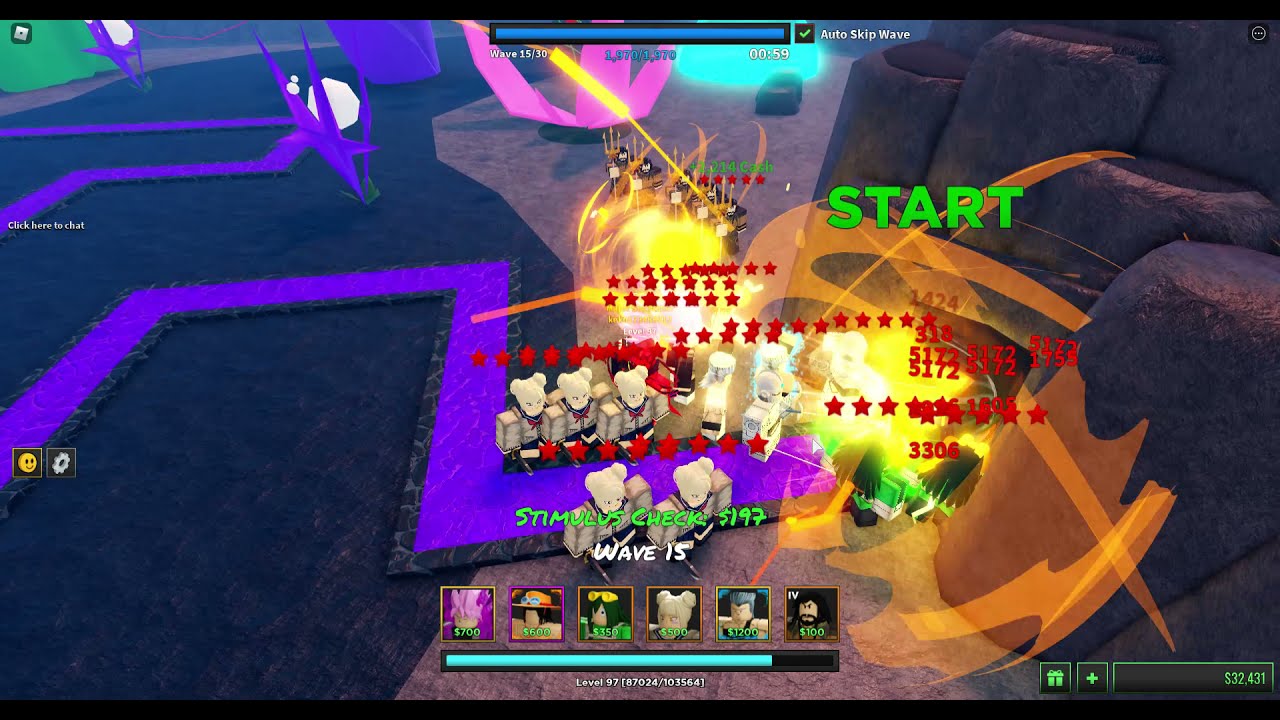The screenshot depicts a top-down action platformer or arena-type video game with various elements presented on a colorful battlefield. At the bottom of the screen, there is a row of six small square icons, each featuring different characters, likely representing the player's team. These characters have numerical values, potentially indicating their health. The player's health bar appears as a steel bar with a portion colored black, suggesting some health is depleted. On the lower right, green text displays the player's money or points.

The main scene showcases numerous squared-off bear-like characters engaging in combat on vibrant platforms, with a prominent purple platform resembling a sideways, squared-off question mark. The characters hurl attacks at one another, causing orange explosions and damage numbers to appear overhead. The background is adorned with purple paths, suggesting additional areas for movement and battle. Surrounding this chaotic scene are bright neon colors, such as pink and blue, and geometric shapes creating a visually striking environment.

On the right side of the image, tall gray mountains and rocks are visible. Text elements are prevalent throughout the screenshot; in the upper right corner, phrases like "auto skip wave" and "start" can be seen in green letters. Red numbers and stars also dot the battleground, signifying some form of scoring or damage indicators. Additionally, the phrase "stimulus check, 197" is displayed in green text, further contributing to the dynamic and detailed interface of the game screen.